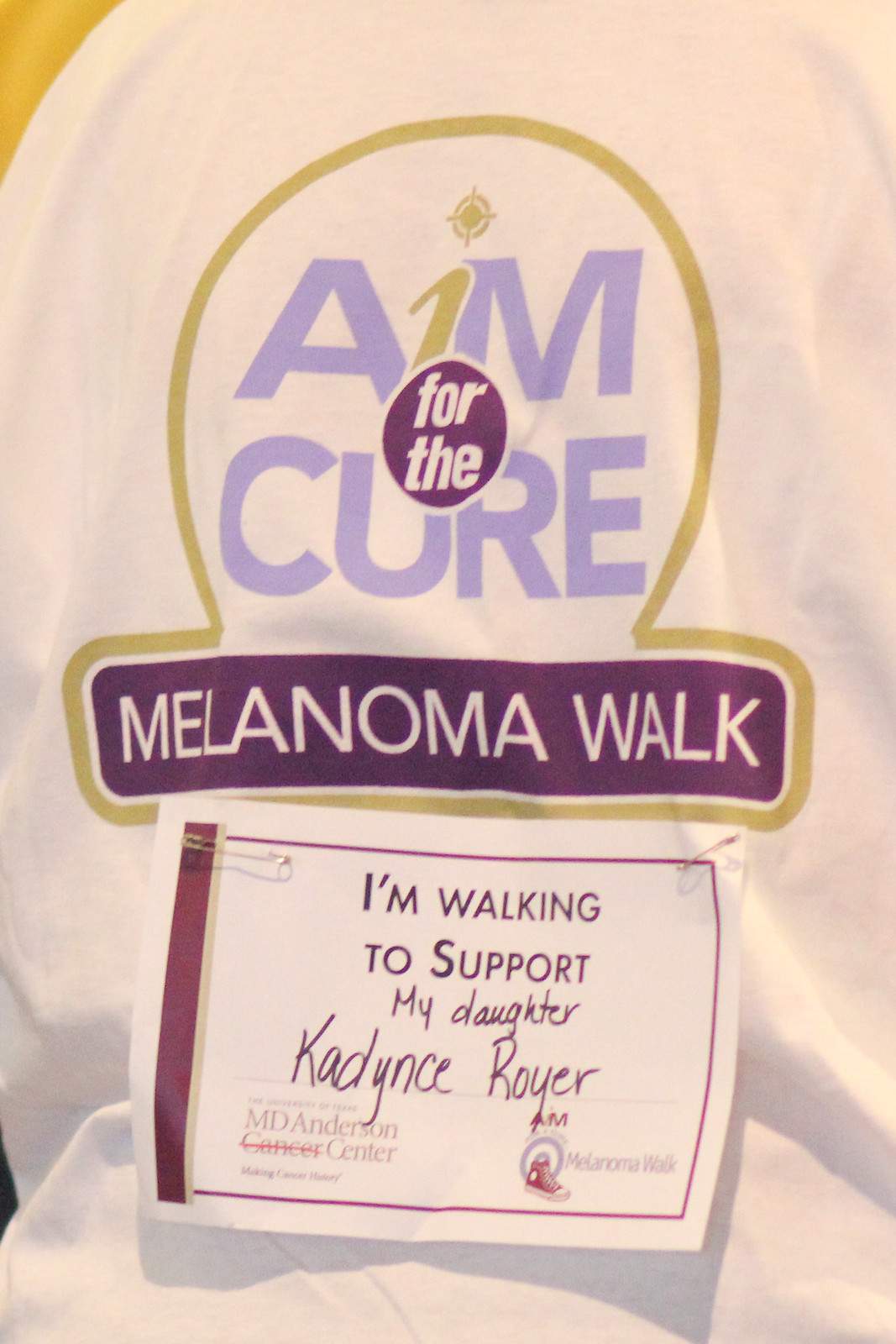The image displays the front of a white t-shirt prominently featuring the phrase "Aim for the Cure" in large letters. The word "Aim" is in blue with the "I" uniquely standing out in yellow and dotted with a yellow period. Positioned below this is "Cure," also in blue letters. Central to this design is a white circle with a black background encapsulating the phrase "for the." Beneath this, "Melanoma Walk" is written horizontally in a dark color. Affixed to the shirt is a piece of paper with a maroon border, bearing the message "I'm walking to support my daughter, Cadence Royer," along with the insignia of the MD Anderson Cancer Center at the bottom right and another logo related to the Melanoma Foundation at the bottom left. The design includes a detailed depiction of logos, with a small circular top-hat-like logo featuring a thin gold border and a signature element of a bullseye serving as the dot in the "I" of "Aim." The comprehensive visual elements and supportive message illustrate a commitment to the melanoma walk event and personal dedication to fighting skin cancer.